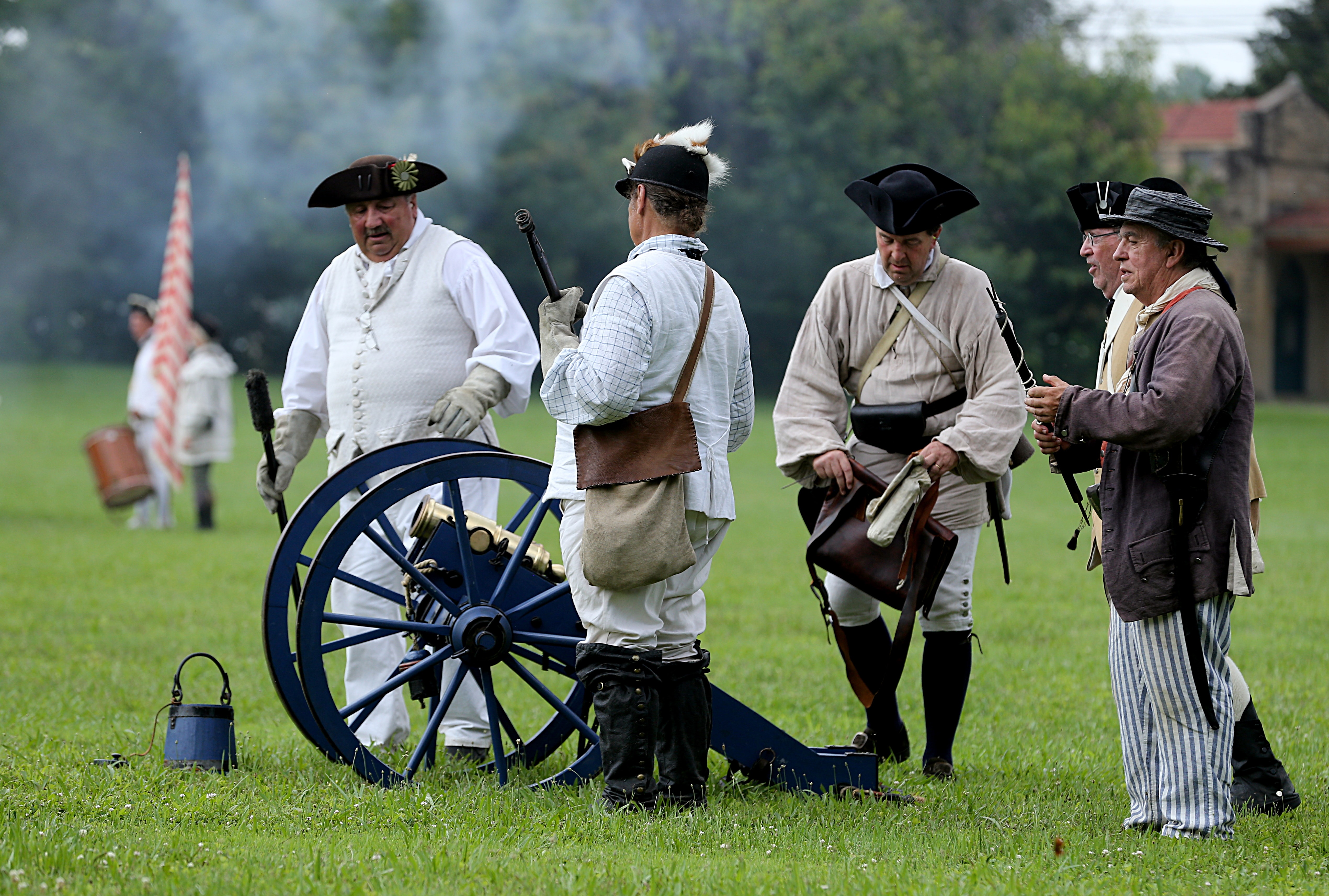This vibrant outdoor photograph captures a detailed historical reenactment of the Revolutionary War in a park setting. At the center, five men are dressed in authentic colonial attire, featuring white and brown outfits with button-up vests and black boots. They don iconic black hats—some tricorn hats and others adorned with feathers, signifying military status. The focal point is a coppery brass cannon mounted on a striking blue chassis with large wheels. The men are actively engaged in the process of loading the cannon, with one man holding a baton to pack the gunpowder. A matching blue pouch is situated nearby, likely containing additional supplies. In the background, trees and a historic building are visible, adding depth to the scene. An American flag held by an individual with a large drum further enhances the authentic ambiance of the reenactment, evoking the spirit of the 1700s Revolutionary War.